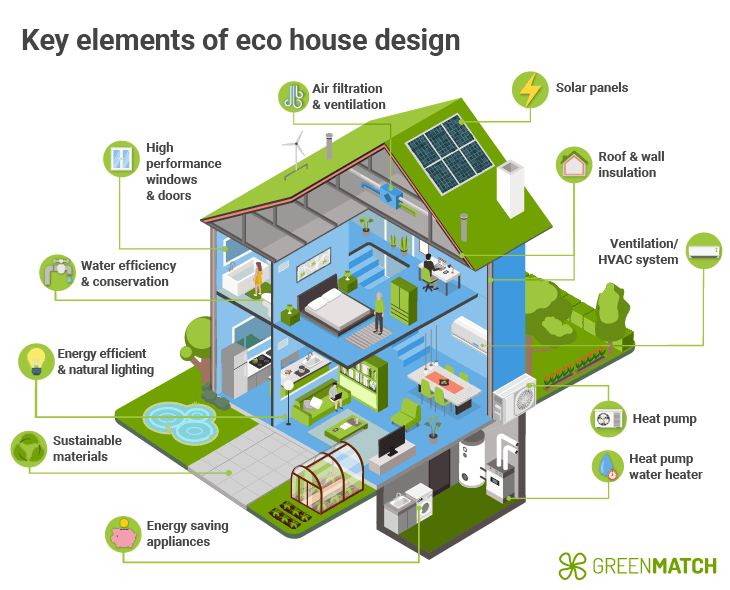The illustration is a detailed cross-section infographic titled "Key Elements of Eco House Design," prominently displayed in bold black text at the top. The digitally rendered, three-dimensional home showcases its green roof and blue walls, with a cutaway view that reveals the various inner rooms and systems spanning from the attic down to a two-story basement. The house is brimming with sustainable, energy-saving features highlighted by small green circles with icons pointing to respective parts of the house.

For example, a lightning bolt icon indicates solar panels situated on the roof. Another icon, a light bulb, points to a lamp inside the house, signifying natural lighting and energy efficiency. Other key features include roof and wall insulation, air filtration, ventilation systems, HVAC, heat pump, and a heat pump water heater, all aimed at maximizing sustainability. 

The overall design emphasizes elements such as sustainable materials, energy-efficient appliances, water conservation, and high-performance windows and doors. The bottom right corner of the infographic features the company logo, "GreenMatch," accompanied by a small green fan icon. Additionally, the house contains people in different rooms, including the kitchen, living room, and bedrooms, illustrating its functional and livable environment.